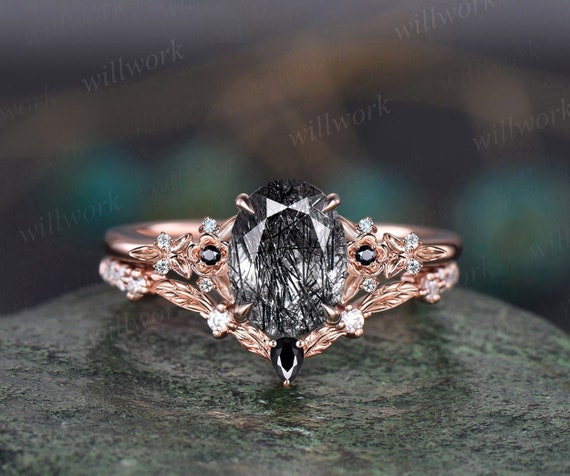The photograph, perfectly square in shape, features a rose gold ring elegantly resting on a dark gray piece of granite rock. The background transitions from a blackish-blue shade at the top to a stone-like texture at the bottom. The ring, designed with two intricately adorned bands, showcases an oval-shaped black charcoal diamond at its center. Surrounding this main gemstone are smaller diamonds, as well as additional black stones that complement the central diamond. The bands of the ring are embellished with delicate floral patterns and tiny diamond studs, and feature fine engravings that resemble feathers. A faint, diagonal text at the top reads "will work." The image's focus is on the exquisite details of the ring, with the background purposefully blurred to enhance its prominence. The design thoughtfully incorporates the reflective qualities of the gemstones, enhancing the allure of the rose gold craftsmanship.